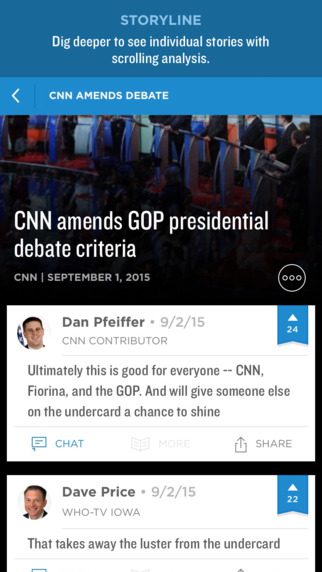Here's the cleaned-up and detailed caption for the image described:

---

The screenshot captures a segment from the CNN mobile app. At the top, a blue header features a light blue storyline titled "Dig Deeper," inviting users to explore individual stories and analysis through scrolling. Just beneath this header, there's a lighter blue banner displaying the text "CNN Amends Debate" alongside a left-pointing arrow.

The background image under the header shows GOP candidates standing at podiums during a debate. Overlaying this photo, white text announces, "CNN Amends GOP Presidential Debate Criteria," with the publication date "CNN September 1st, 2015" positioned below.

In the bottom right corner of the image is a circular icon containing ellipses. Below the main image, two white boxes are visible. The top box mimics a tweet, attributed to Dan Pfeiffer, with his profile photo on the top left and his name, a date, and his designation as a CNN contributor on the right. A blue bookmark icon on the far right of the box indicates that 24 people have bookmarked this item. The message content follows this header, and at the bottom of the box, options to "Chat" and "Share" are placed on the left and right, respectively.